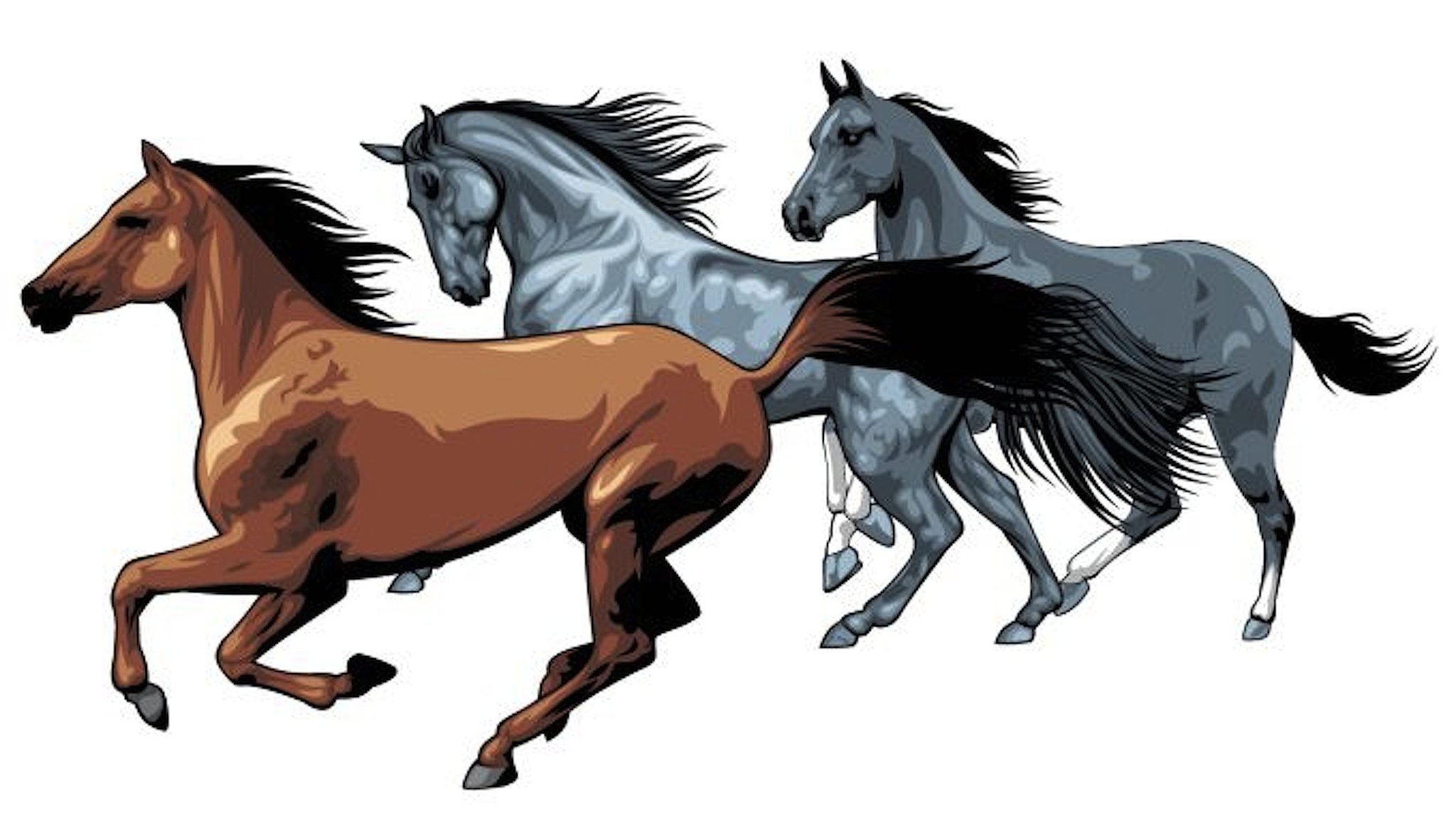This is a highly detailed digital artwork depicting three galloping horses on a pure white background, giving the impression of a vibrant equestrian scene. The horses are running from right to left, all positioned in profile view. Leading the trio is a brown horse with a black mane and tail. Its front hooves are raised high in the air, capturing the motion of its full gallop. Behind it, a dappled gray horse follows closely, also in mid-gallop. This horse features a black mane and tail, and its head and neck are tucked down towards its chest, enhancing the dynamism of its movement. The last horse, slightly trailing, is a darker bluish-gray dappled horse. It has distinct black mane and tail with white markings just above its hooves, and its ears are perked up as it runs. All three horses are detailed meticulously, showing lifelike anatomy and fluid motion, making the scene vivid and engaging. There are no other elements or text in the image, focusing attention entirely on the majestic galloping horses.